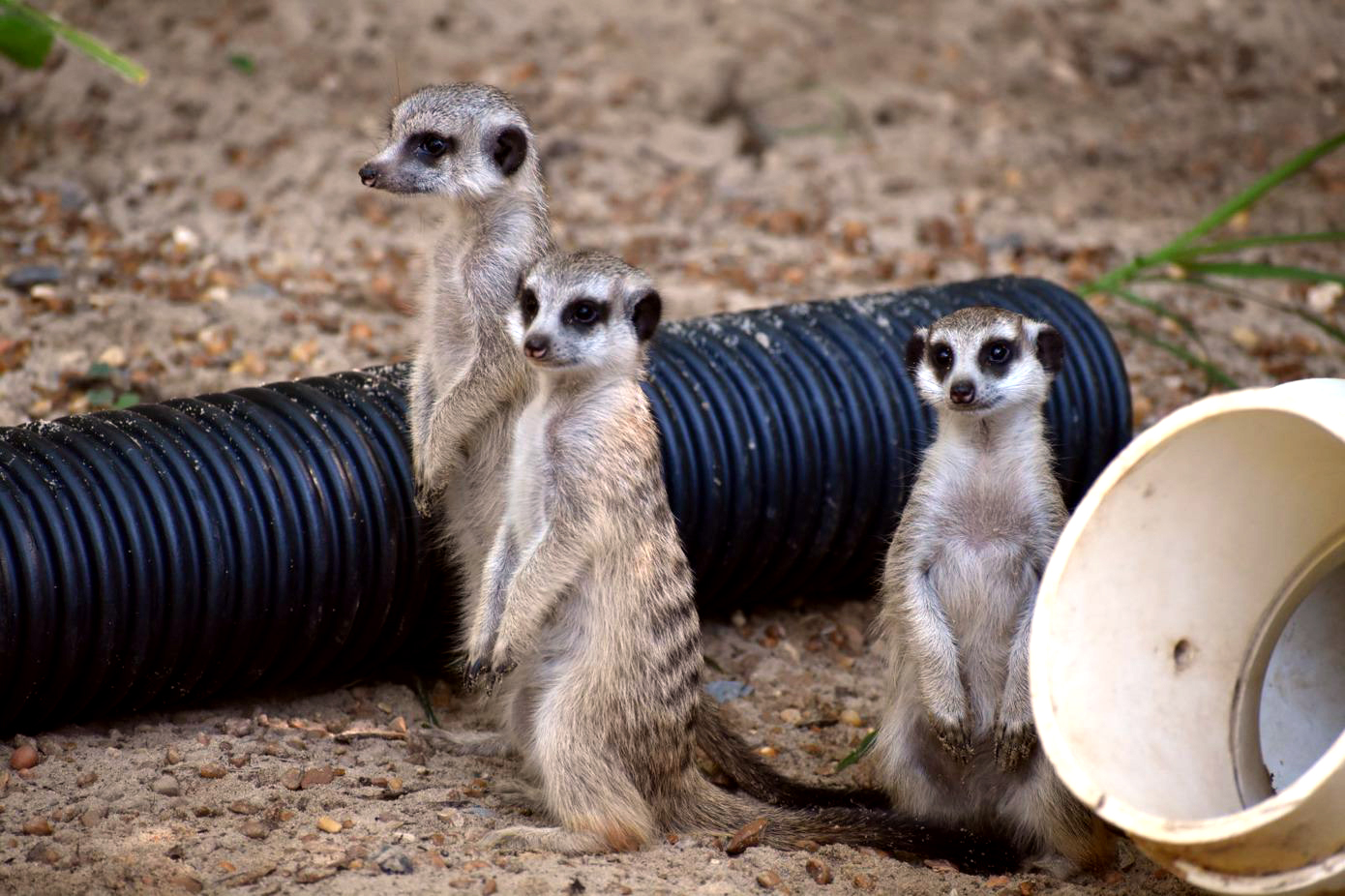The photograph depicts three small mammals, likely meerkats, standing upright on their hind legs on a sandy, rocky ground. They have distinct black markings around their eyes, giving them a panda-like appearance, with small, black ears and long, dark brown tails. Their noses and the insides of their ears are also black, contrasting with their off-white, almost brown bellies and faces. Behind them lies a coiled black PVC pipe, possibly a part of their habitat or a play toy, hinting that they might be in a controlled environment like a zoo. The surroundings include some green plants and a mix of dirt and loose soil. Two of the meerkats are looking off to the left side of the photo, while the third one stares directly ahead, adding a dynamic sense of vigilance and curiosity to the scene.